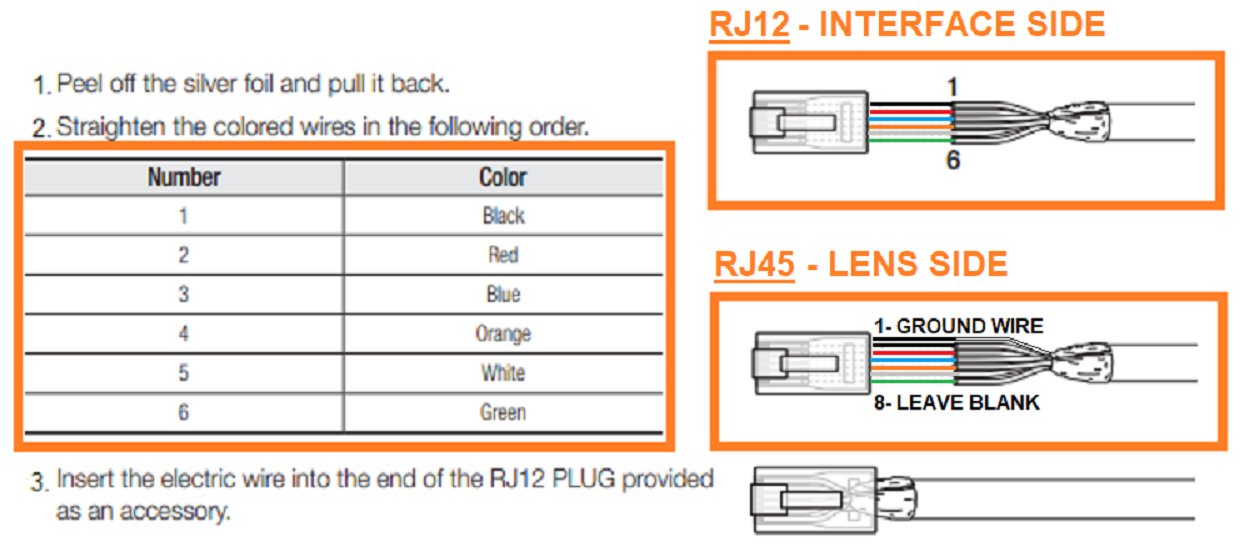This detailed instructional image guides the user on assembling an electrical RJ12 connector. On the top left, against a white background with black text, steps one through three are listed for clarity. Step one instructs to peel off the silver foil and pull it back. Step two states to straighten the colored wires in the specified sequence: a chart bordered in orange details the order—Number 1: Black, Number 2: Red, Number 3: Blue, Number 4: Orange, Number 5: White, and Number 6: Green. Step three directs inserting the electric wire into the RJ12 plug, provided as an accessory.

To the right, the image includes a diagram labeled "RJ12 interface side" on an orange background, illustrating the plug and the color-coded wires. Below this, another diagram titled "RJ45 lens side" (also on an orange background) shows the configuration, specifying the ground wire (position 1) and a blank space (position 8). At the bottom, the completed assembly of the wire is depicted, providing a comprehensive visual guide for the wiring process.